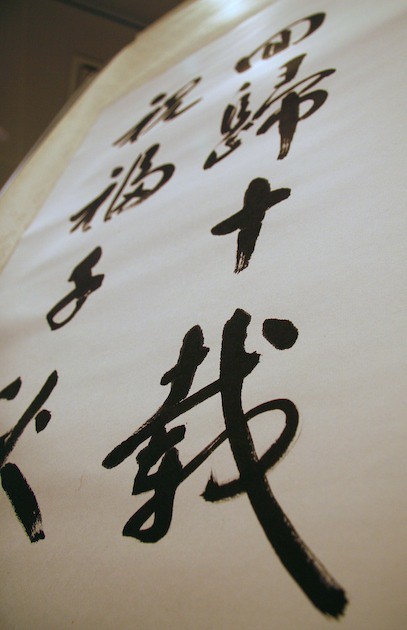The image showcases a traditional Asian scroll, possibly featuring Chinese or Japanese calligraphy, mounted on a tan-colored wall. The scroll has a mostly white background that appears slightly tan towards the bottom due to shadowing, suggesting the photo was taken from the ground floor looking upwards. The black calligraphic characters, painted with a wide brush, stand out prominently against the white, parchment-like surface of the scroll. The top left corner reveals a section of the beige wall which exhibits some distortion and blurriness. Overall, the setting is well-lit, providing clear visibility of the scroll and the wall, and a brown trim is visible near the ceiling in the back left corner of the image.